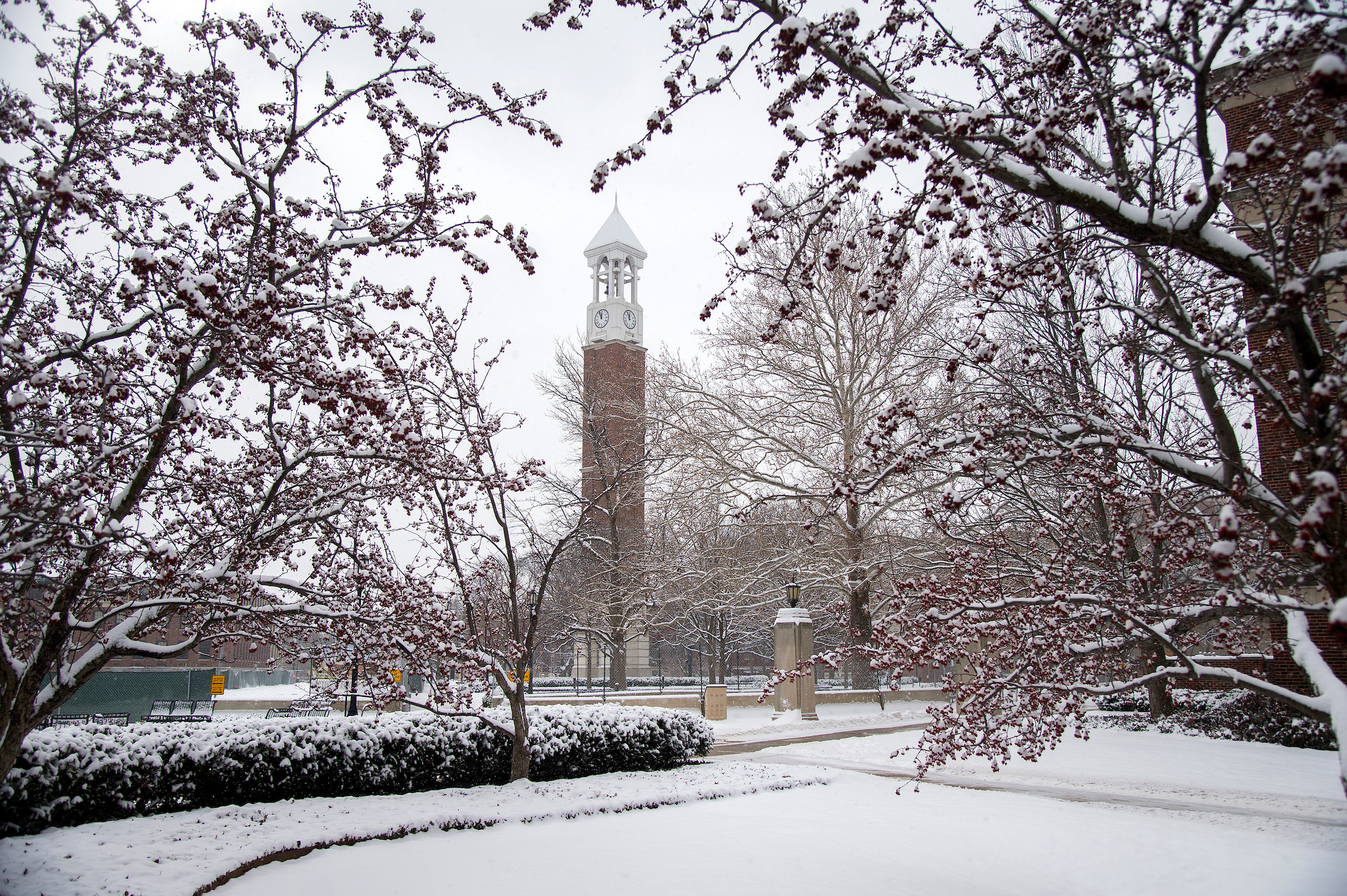Amidst a tranquil snowy landscape under a white, cloud-filled sky, the focal point is a tall, red brick clock tower, its upper section transitioning to a white structure with a pointed spire. Beneath the spire, arched openings reveal a bell, framed by clocks on each side. Framing the scene, snow-laden branches and shrubs with red berries lead the eye toward the tower. The foreground features a brown pathway winding through the snowy terrain. To the left, a green fenced area and a red building can be seen, while to the right, a dark, red-bricked building stands behind trees with snow-laden branches, possibly bearing small pink or reddish leaves. Additional surroundings include lantern-adorned stone structures and snow-covered benches, capturing the serene essence of this winter scene.